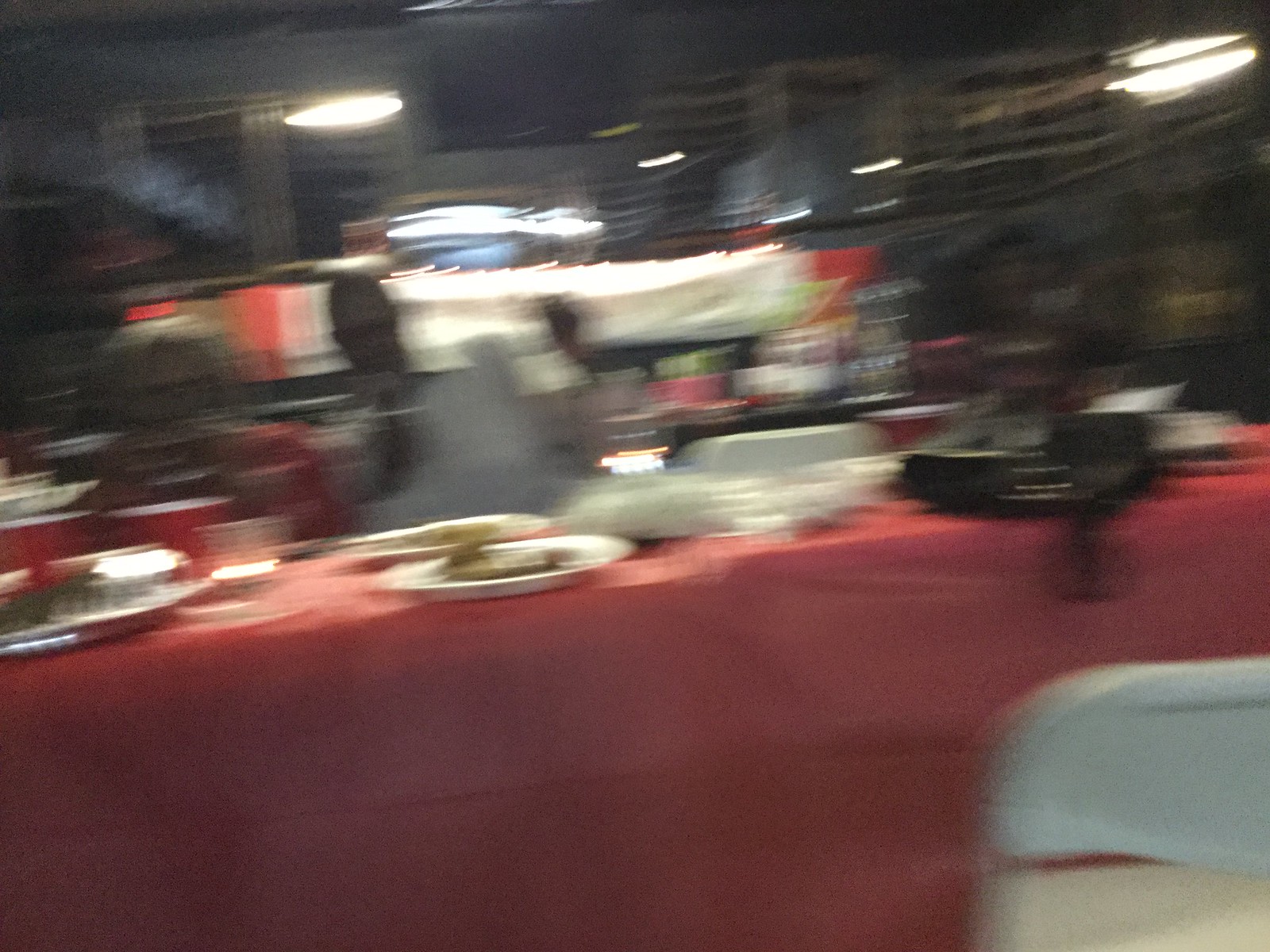The image depicts a dimly lit indoor setting, possibly a basement or restaurant, hosting a banquet with numerous dishes spread across a long table adorned in a red plastic tablecloth that extends to the ground. Despite the heavy motion blur, white and black plates can be discerned among the varied assortment of food. Notable red and translucent cups are placed alongside the dishes, which include beige and red food items. There's a mix of folding and possibly upholstered chairs, with one particularly prominent on the lower right side of the image. The background reveals ceiling lights, faint shelf-like structures, and potential reflections suggesting a complex, yet indistinct environment. Additionally, a mysterious black object with a cord, possibly an old telephone or till, is visible on the right side of the table. To the left, a staircase might be perceived, further indicating the diverse elements within this convivial, albeit blurry, scene.